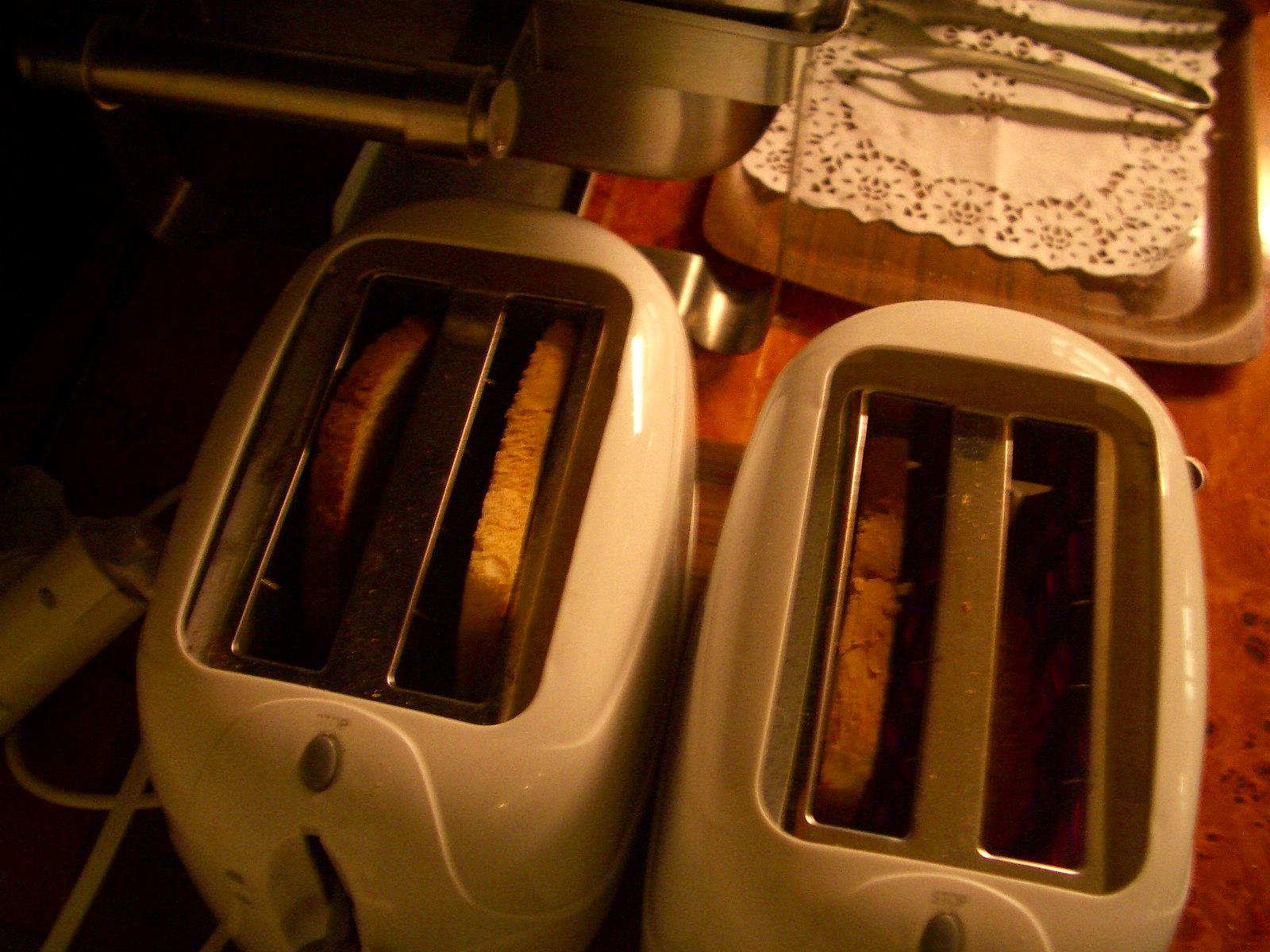This is a color photograph taken from above, depicting two side-by-side, cream-colored toasters on a red surface. The toaster on the left contains two slices of bread, while the toaster on the right has one slice. Both toasters have gray "stop" buttons at the top and levers for lowering the bread. The scene is somewhat shadowy, particularly on the left side, and is tinged with a brownish filter, making the true colors slightly ambiguous. Behind the toasters, in the upper right corner of the image, there is a wooden tray adorned with a white lace doily. On the tray rests a pair of metal tongs. A power cord is visible extending from the left toaster. Additionally, a shiny metal object and another piece of equipment can be seen near the back of the first toaster. The overall composition suggests a setting where breakfast is being prepared.